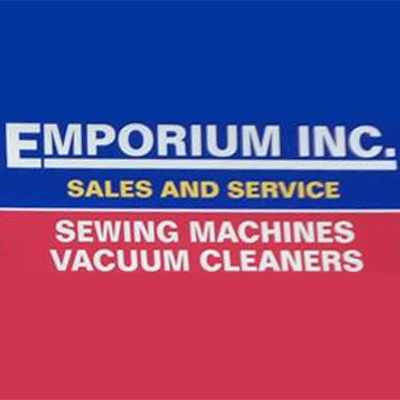The image depicts a square, vertical, and rectangular business advertisement sign for Emporium Incorporated. The top half of the sign features a blue background with the company name, "EMPORIUM INCORPORATED," written in all-cap white text. A white line extends from the first "E" across the rest of the words. Below this, "SALES AND SERVICE" is prominently displayed in yellow, all-caps text against the same blue background. Separating the top and bottom halves of the sign is a horizontal white stripe. The bottom half of the sign has a red background with two lines of text in all-caps white letters: "SEWING MACHINES" on the first line and "VACUUM CLEANERS" directly underneath it. The colors of the sign are somewhat faded and dull, and the text appears slightly blurry but remains readable.